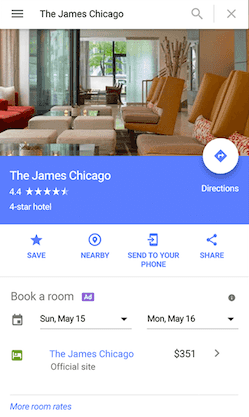The image depicts a search result page for "D. James Chicago." The top section features a white search bar with the query "D. James Chicago" inside. To the left of the search bar is a menu icon, and to the right is a close icon, both in black. 

In the main section of the page, there is an image showcasing the interior of a hotel. The hotel features brown sofas on the right side and red sofas on the left side. White tables are scattered throughout, and large windows adorn the walls. The right-side wall is painted yellow.

Below the hotel image, a blue background features white text stating "D. James Chicago, 4.4 star rated," indicating it is a 4-star hotel. To the right, there is a button labeled "Directions."

At the bottom of the page are four blue buttons: "Save" on the left, followed by "Nearby," "Send to Your Phone," and "Share" on the right.

Additional text at the bottom mentions booking details: checking in on Sunday, May 15, and checking out on Monday, May 16. Underneath, it mentions the "D. James Chicago official website," with an icon of a bird on a green background to the left. The price listed is $351, located on the right. Lastly, "more room rates" is an option in blue text on the bottom left.

The overall background of the image is white, except for the blue backdrop underneath the hotel photo.